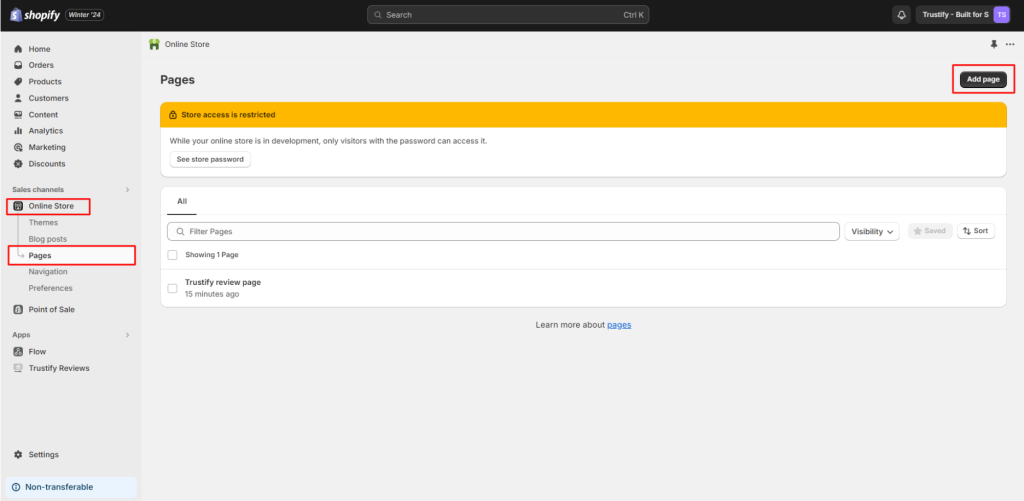Screenshot from Shopify Admin Dashboard Detailing the Online Store Setup:

The screenshot showcases a section of the Shopify admin dashboard, predominantly set against a white background. On the left panel with a gray background, the following menu options are listed vertically: Home, Orders, Products, Customers, Content, Analytics, Marketing, Discounts, Basic Channels, with a red square highlighting "Online Store", followed by Themes, Blog Posts, and Pages, each circumscribed with a red outline. Further down, Navigation, Preferences, Fonts, and Apps for Flow and Yotpo Reviews are visible. Below these options, there is a "Settings" tab, accompanied by a small blue box labeled "Non-Transferable."

On the main section under the header "Online Store," there is a notification in an orange box stating, "Store Access is Restricted." It specifies, "Your online store is in development, only visitors with a passcode can access it," followed by an option to "See Store Password." Below this, a white box is titled "All," indicating it is currently selected, with a gray outlined box labeled "Filter Pages." Subsequently, it states, "Sharing One Page" and lists "Trustify Review Page." To the right of the Filter Pages box, options for "Visibility" and "Fonts" are mentioned. At the bottom of this section, there is a link prompting users to "Learn More About Pages."

The layout and highlighted sections indicate areas the user may need to configure, especially focusing on the development status and restricted access of the online store.